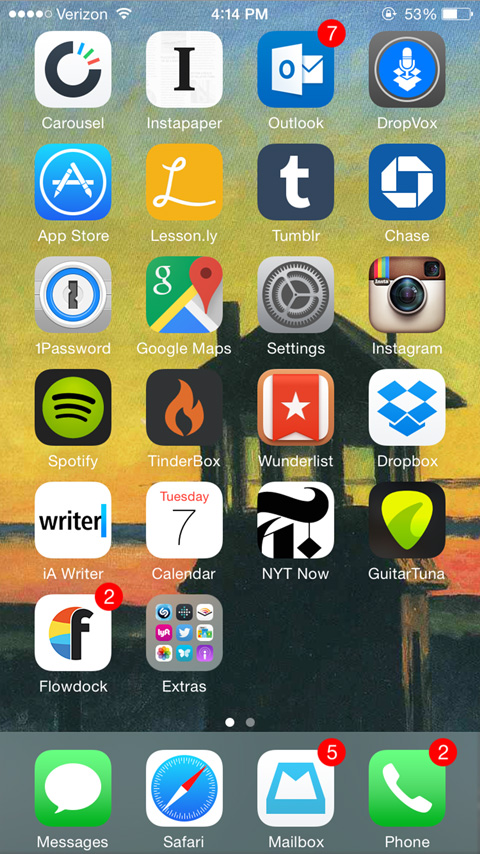The screenshot depicts an iPhone home screen featuring a detailed and visually captivating wallpaper. The background showcases a narrow and small tree house or guard house with an angled roof, set against the vibrant hues of a sunset. The icons on the home screen are neatly arranged in rows of four, with the exception of the last row, which contains only two icons. 

In the bottom section of the screen is the phone's control panel. The bottom left corner displays the Messages app, followed by Safari, then the Mail app, which has a red circle in the top right indicating five unread emails. To the right of Mail is the Phone app, which also shows a red circle with a number two, signifying two unread messages or missed calls.

The top left corner hosts the Carousel app, followed by Instapaper, Outlook, and Dropbox. The subsequent icons include the App Store, Lesson.ly, Tumblr, Chase Banking App, 1Password, Google Maps, Settings, Instagram, Spotify, Tinderbox, Wunderlist, Dropbox (appearing again), Writer, Calendar, New York Times Now, Guitar Tuna, FlowDock (which has two alerts), and lastly, a folder labeled “Extras” that contains nine additional app thumbnails.